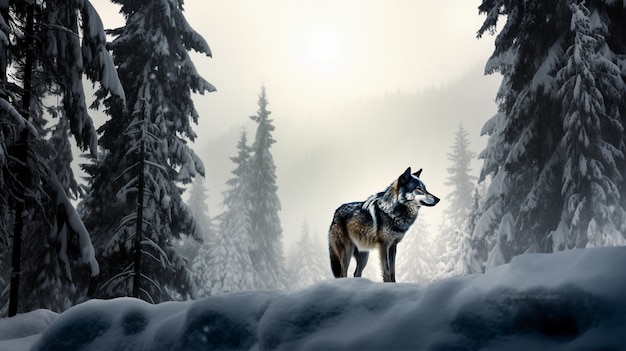In this detailed image, a lone wolf with thick, multicolored fur—ranging from black and brown to white and gray—stands at the center of a snowy, high-altitude winter forest. The setting features a clearing surrounded by tall, snow-laden alpine trees, their branches heavy with a thick layer of snow. The scene is characterized by its gray, hazy atmosphere, with feeble sunlight attempting to pierce through the overcast sky, casting a muted glow on the shimmering snow. In the background, the silhouette of a majestic mountain rises, adding depth and scale to the image. The wolf, with its ears pointed and eyes gazing calmly to the right, exudes a serene and observant presence against the tranquil and somber landscape.